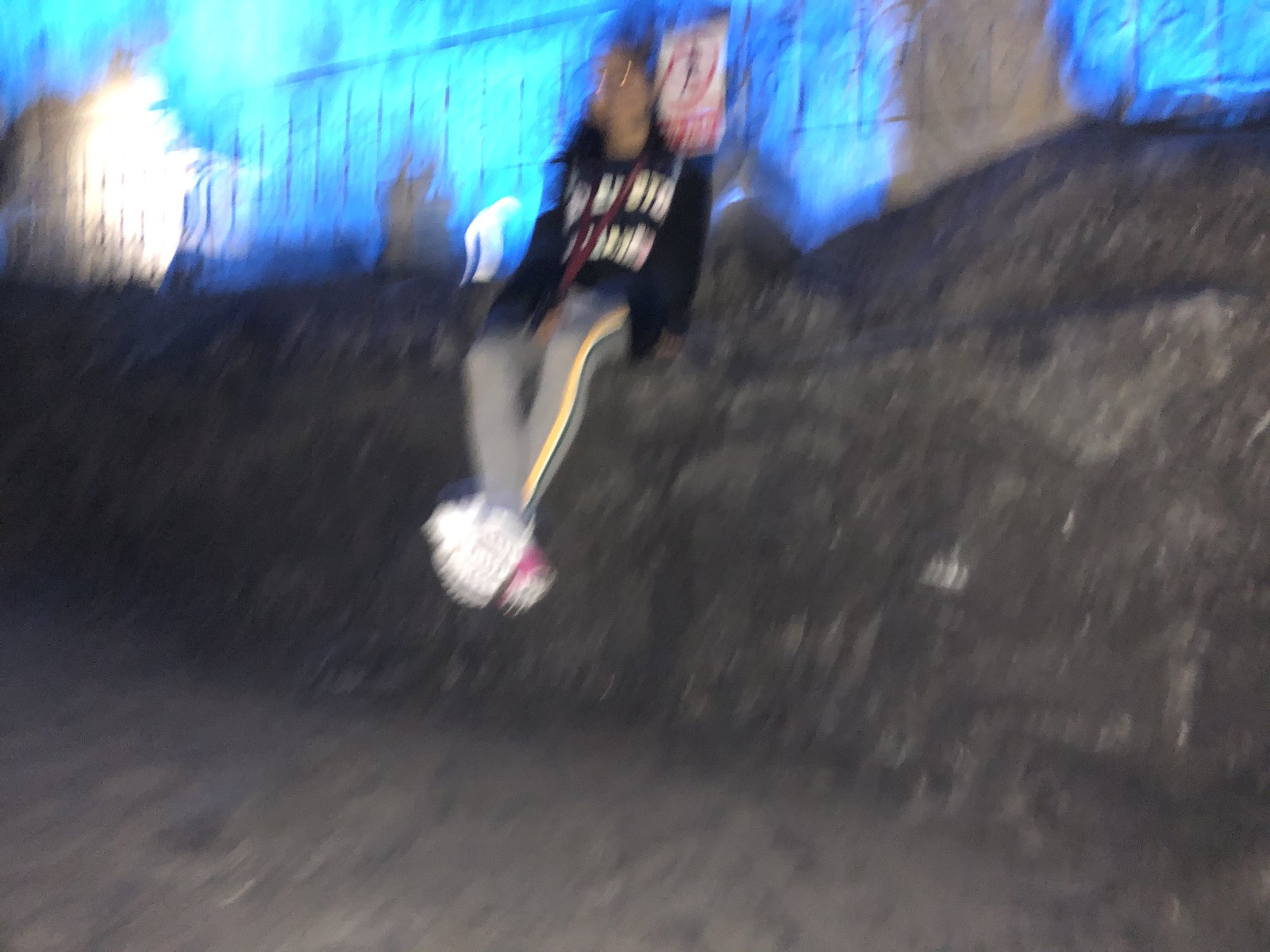A blurry photograph captures a young girl sitting on a gray, rock-stone wall in a graveyard. She is casually perched on the approximately four-foot-tall wall, which has a metal slat fence on top. The ground below the wall appears gray, suggesting a stone path. The girl is dressed in gray leggings with a striped pattern featuring yellow, white, and black, and her ankles are crossed, revealing white and pink sneakers. She wears a black hoodie with indiscernible white lettering and has a burgundy lanyard slung across her shoulder next to a satchel on her right side. In the background, a red and white sign is faintly visible. Overall, the girl appears to be relaxing in this serene yet somber setting.